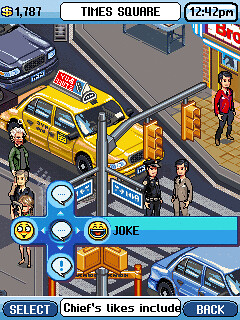The image is a screen capture from a mobile game set in an urban environment resembling Times Square. It is depicted in pixel art and displayed in vertical portrait mode. At the top of the screen, there is a blue bar showing a dollar amount of $1,787 in yellow, the text "Times Square" in the center, and the time "12:42 p.m." on the right. Below this, the interactive interface includes a four-way controller featuring two emojis: a suspicious-looking face and a laughing face with the word "joke" beneath it. Additional icons include a chat bubble and an instructional exclamation mark bubble.

In the central section of the image, various urban elements are detailed. A yellow taxi with a sign on top and text on its side is seen on the gray road. Nearby, a police officer is talking to a person in a business suit. On the right, a person with black hair is walking, dressed in a red suit jacket, black pants, and brown shoes, with red and brown text above him. The street scene also includes a man holding a camera on the left, another person holding a cell phone, and multiple cars—including a blue car and a gray car. A traffic light extends from a metal pole in the middle of the scene.

The lower part of the screen displays options such as "Select" on the left, "Back" on the right, and a white bubble reading "Chief's Likes Include" at the bottom center, though the text is cut off. The surrounding environment features the busy ambiance of a city intersection, emphasizing the dynamic and vibrant atmosphere reminiscent of Times Square.